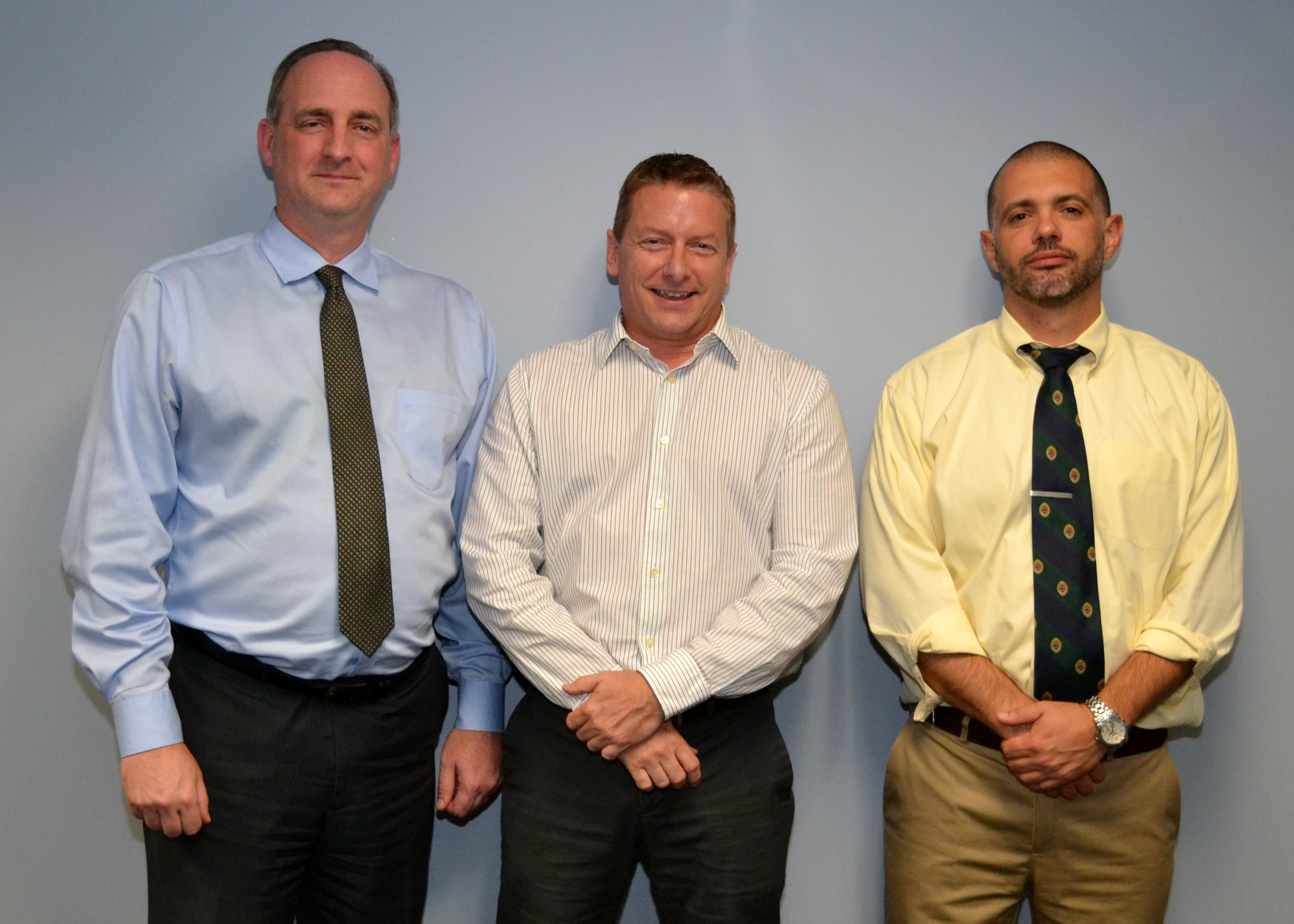The image features three professionally dressed Caucasian gentlemen standing shoulder to shoulder against a pale blue backdrop. From left to right: the first gentleman is the tallest, sporting a light blue button-up shirt paired with a dark yellow-black tie and black trousers. He stands with his arms hanging down by his sides, showcasing short darkish, almost greying hair and a subtle smile. The middle gentleman, shorter in stature, wears a white striped button-up shirt with the top button open and gray slacks. He has light brown hair and a big smile, revealing his teeth, while he keeps his arms crossed in front of him. The third gentleman has light brown, shaved hair with a beard, and is dressed in a yellow button-up shirt, a black tie adorned with yellow dots and hints of red, and khaki-colored trousers. He stands with his arms crossed, revealing a watch on his left wrist, sporting a neutral, composed expression.